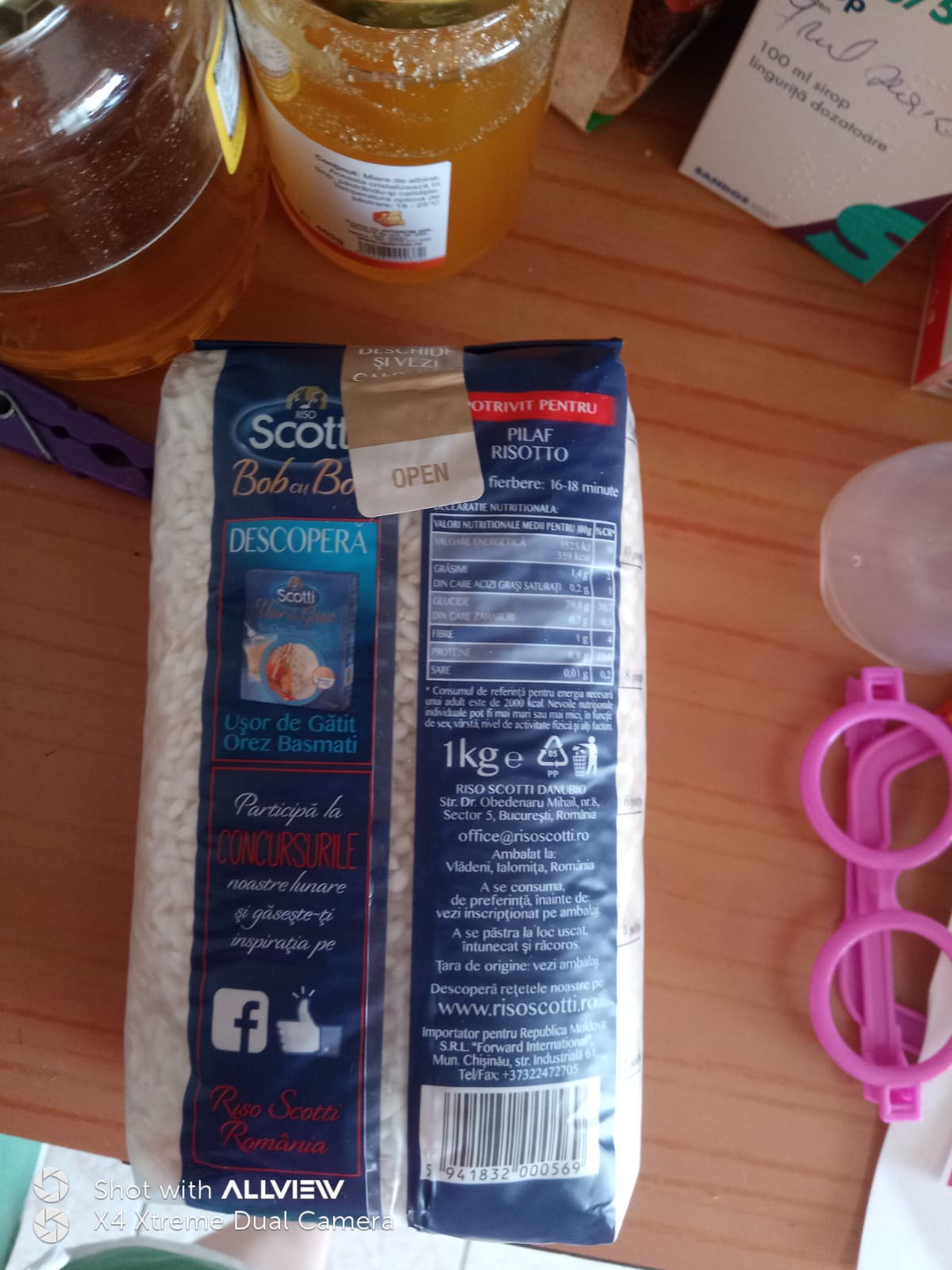A bag of risotto lays face down on a wooden tabletop, prominently displaying its dark blue nutritional label and barcode. The top of the bag features a gold and white resealable tape for easy closure once opened. In the upper left corner of the image, two jars rest on the table: one appears to contain apple juice, which is about one-quarter empty, while the other holds an orange liquid or jelly. Underneath the apple juice jar lies a dark blue clothespin. To the right of the risotto bag, a pair of round, pink plastic child’s eyeglasses have been placed. Above the glasses, a white glass can be seen. In the upper right corner, a white box is visible, marked with a blue diagonal section in the lower right corner, which features a green 'S'.